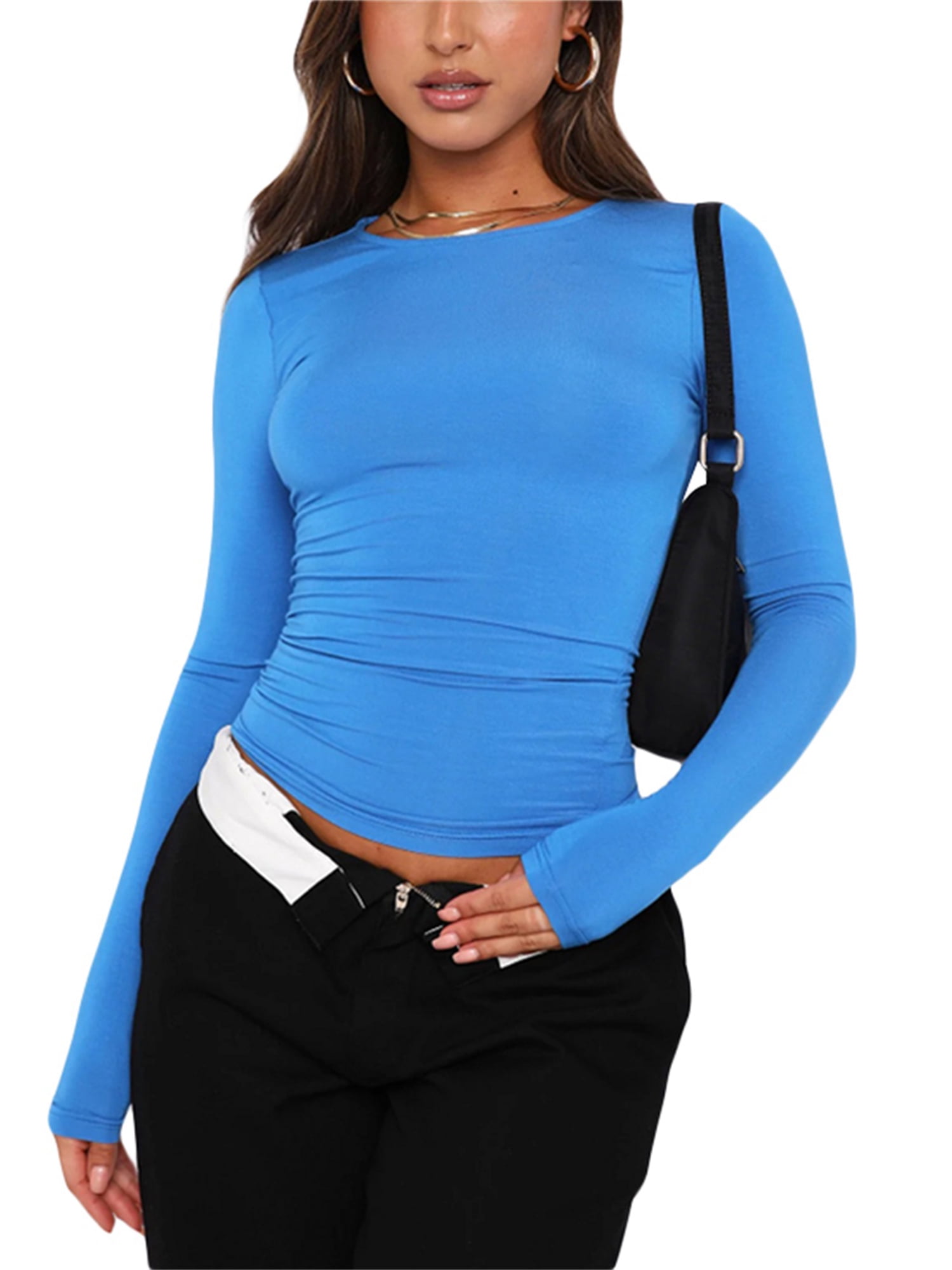In this detailed product photo set against a white background, we see a young woman from just below the eyes to her upper thighs. She has shoulder-length brown hair and a glossy pink lipstick. Her olive skin is complemented by gold hoop earrings and two thin gold necklaces. She is wearing a form-fitting, long-sleeved blue top that extends slightly past her wrists, partially covering her hands which are adorned with peach-colored acrylic nails. Her left hand rests on her waist, while her right hand hangs by her side. The black pants she is wearing are rolled down at the waist, exposing the white inner lining and an unzipped zipper which reveals a glimpse of her midriff. A black purse with a metal buckle is slung over her left shoulder.